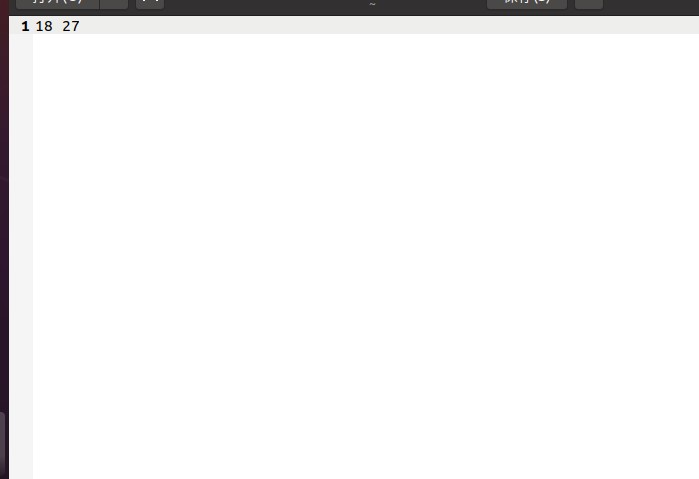The image portrays a zoomed-in view of a foreign text editing program or an editor interface, possibly from a Mandarin-speaking environment. The top section of the interface features a black bar with gray buttons, partially displaying what appears to be Mandarin characters. Because the view is closely cropped and some of the interface is cut off, it is challenging to determine the precise nature of the software.

In the visible portion of the document, a bold number "1" is seen, followed by the numbers "18" and "27." Below these numbers, there is a thin gray bar that outlines the top and edges of the blank, white document interface. The stark white page suggests the document is currently empty. The interface could belong to various types of programs, such as a text editor for writing, a coding environment, or perhaps a mathematical computation tool. Due to the limited and zoomed-in view, it is not possible to specify further.